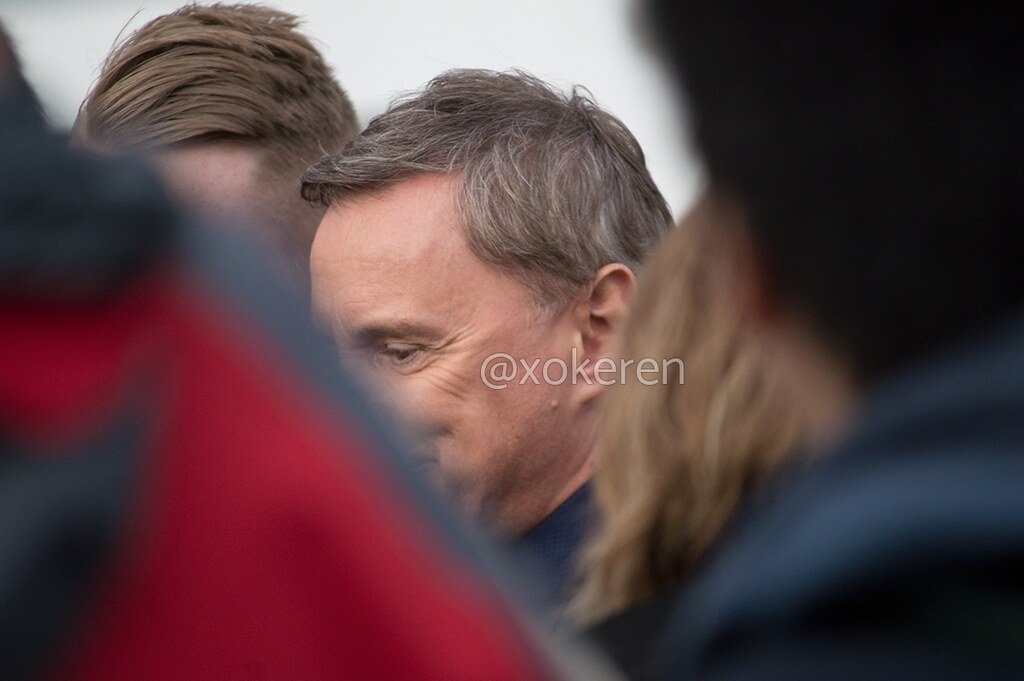The image captures a somewhat chaotic outdoor scene with an overlay watermark reading "@xokeren" in lowercase across the center. The foreground is notably out of focus, as multiple individuals partially obstruct the view. On the left and right edges, there are blurry shoulders of people dressed in raincoats, adding to the obscured and crowded feel. Dominantly, the image centers around an older man who is the most detailed subject, albeit his face is partially blocked by another person in front of him. The older man has short, dark hair with significant gray, suggesting his advanced age, and is looking downward. His expression appears to be a subtle smile.

To his right, the back of a woman's head with blonde, wavy hair is noticeable, although she remains mostly out of focus. Behind her, another man, albeit rather obscured, is discernible by his silhouette; he has black hair and is wearing a black coat. Adding to this clustered scene, there is also a man in a dark jacket with brown hair directly in front of the older man. In another part of the photo, particularly noticeable is a person in a distinctive red and black jacket.

Altogether, the image presents an abstract and layered scene, primarily highlighting an elderly man amidst a bustling, blurred crowd.